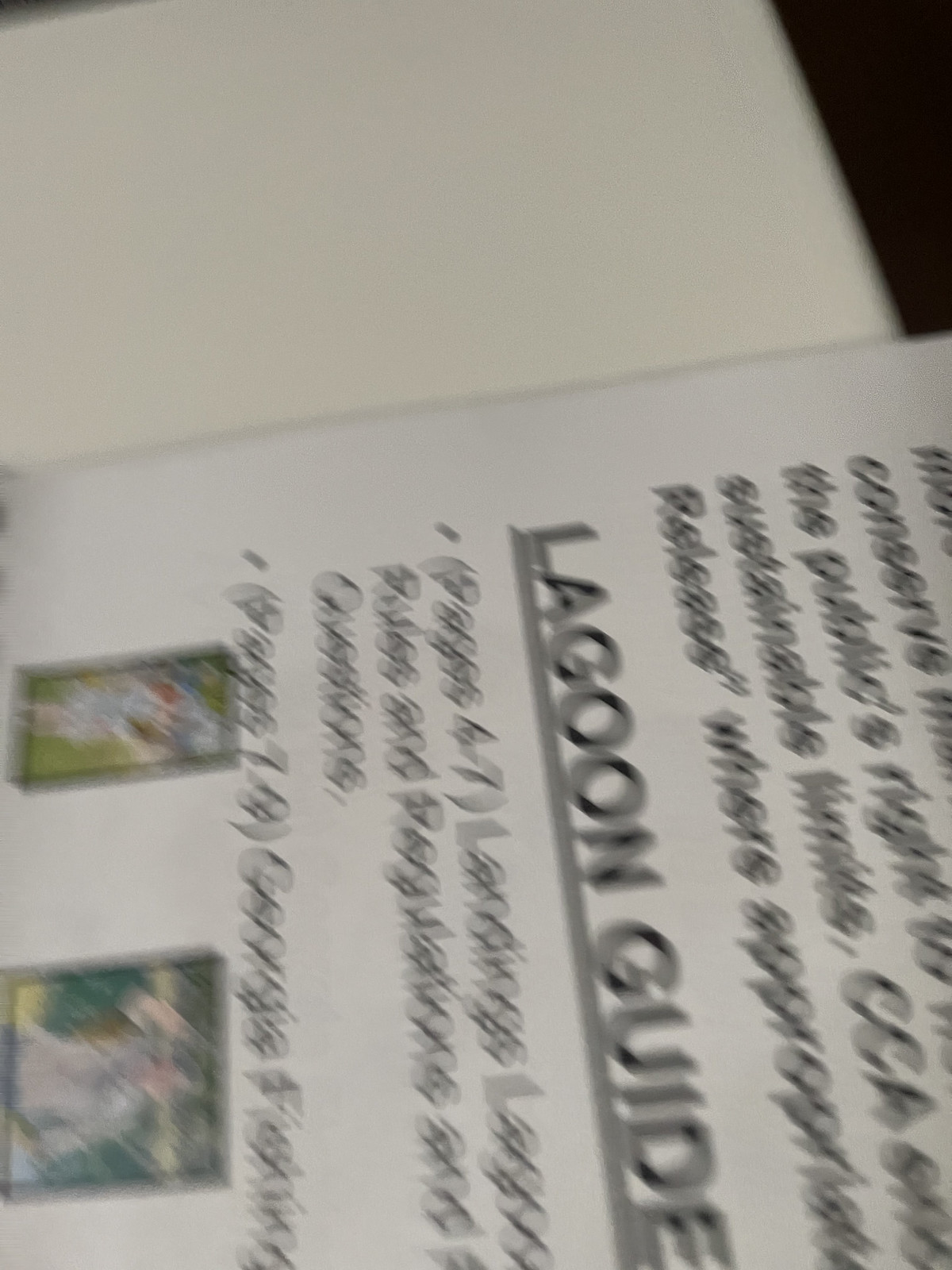The image is a photograph of a blurry piece of paper laying horizontally on a white table. The paper has a white background and prominently features the words "LAGOON GUIDE" in capital black letters at the top. Underneath this title, several bullet points can be made out, though they are somewhat fuzzy. The readable text includes phrases like "The Public's Right To," "Sustainable," "CCA Release Where Appropriate," "Pages 4-7," "Landings Lagoon Rules and Regulations," "Questions," and "Pages 7-9 Georgia Fishing." The bottom portion of the paper contains two rectangular images with colors ranging from light blue to green, yellow, and white, though their details are indistinguishable. The paper is tilted, making it necessary to tilt one's head to the right to read the text.